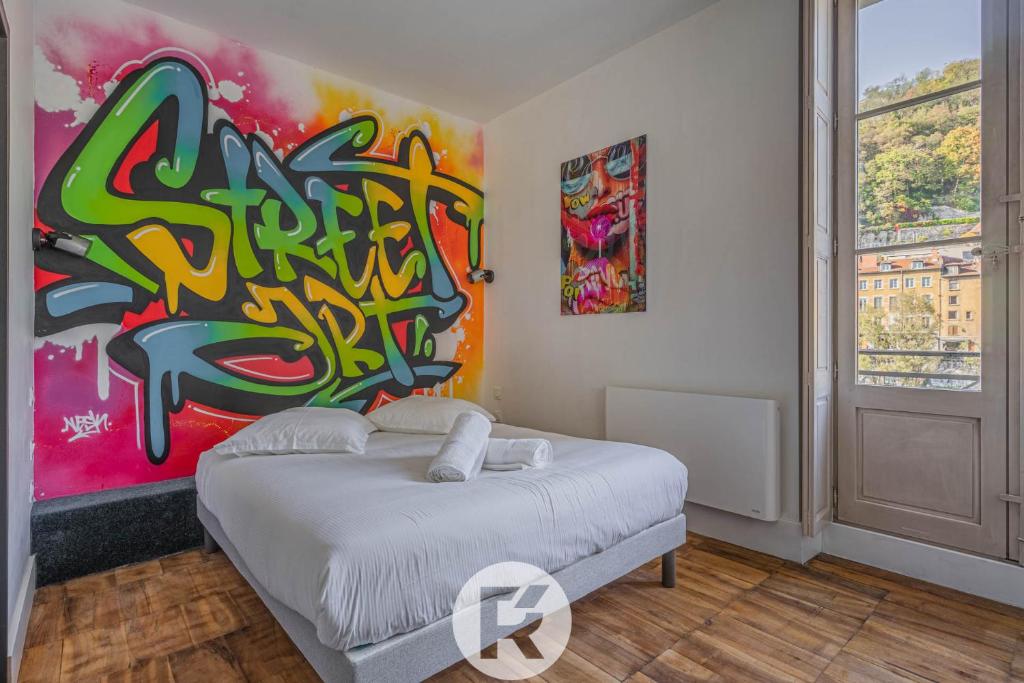This color photograph captures a bedroom with a striking contrast between serene elements and vibrant artwork. The room features a hardwood floor with a neatly made bed draped in white sheets, accompanied by two white pillows and two white towels rolled up on top. Dominating the back wall is an expansive piece of street art, characterized by bold graffiti-style lettering that reads "street art." The mural bursts with vivid neon colors, including green, blue, and yellow, accented by flashes of pink and orange. To the right of this large artwork, there's a smaller poster showcasing a girl's face, adorned with sunglasses and holding a lollipop, rendered in a similarly vibrant graffiti style. This piece complements the larger mural with its colorful mix of pink, orange, and matching tones. The wooden exit door can be seen on the far right of the room. Through a large window on the right-hand side of the photograph, one can view an urban cityscape filled with apartment buildings and trees, under a clear blue sky. The rest of the room maintains a tranquil aesthetic with its white walls, providing an intriguing juxtaposition to the energetic art pieces.